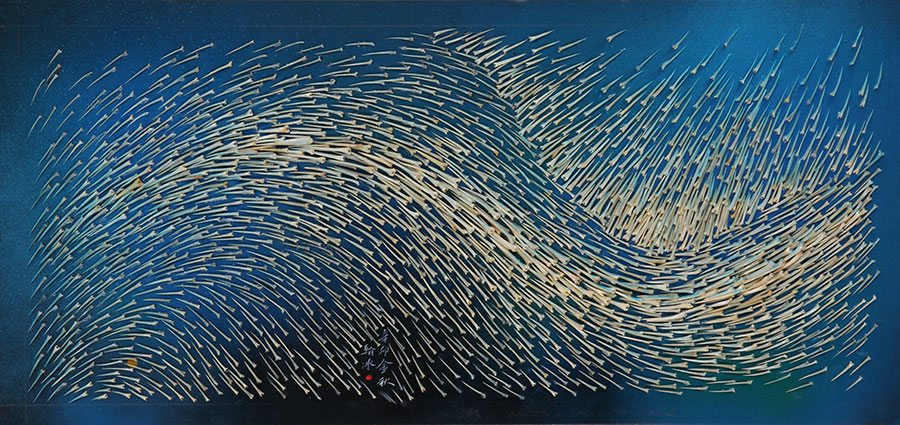The abstract artwork features a predominantly dark blue background interspersed with white, silver, and light blue lines and specks. These elements converge densely in the center, forming a wave-like pattern that undulates across the canvas. The intricate formations resemble the emergent behavior of a swarm, akin to how a school of fish or a flock of birds might move in unison. Additionally, the artwork includes subtle yellowish accents, adding depth and complexity. In the upper right corner, lines appear to counter or press down on the central wave, enhancing the dynamic nature of the composition. Centrally located, there seems to be a signature or writing in Asian script, contributing an additional layer of intrigue to this compelling piece.